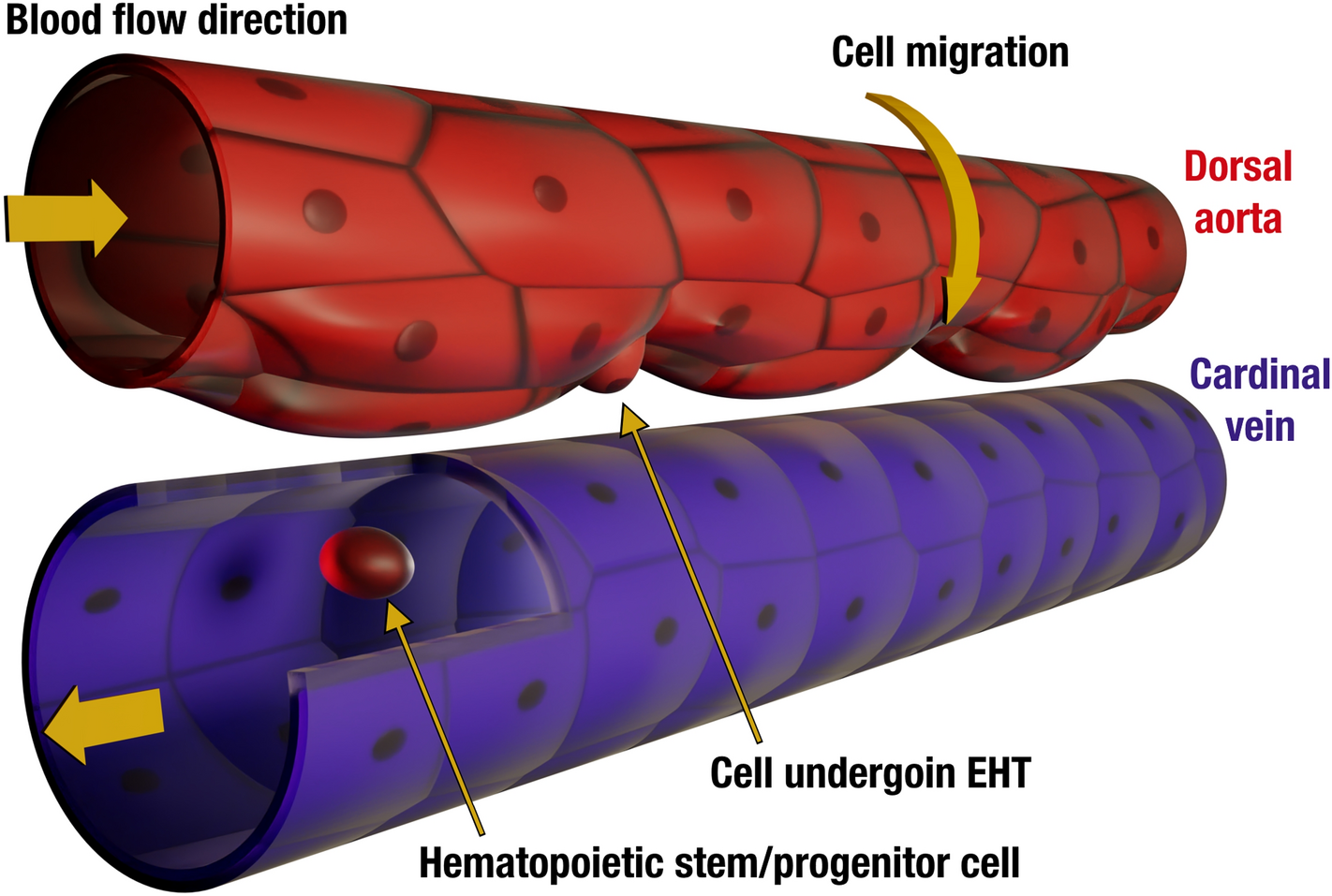This detailed diagram of human blood vessels illustrates two primary structures: the **dorsal aorta** and the **cardinal vein**. The top portion features a cylindrical illustration representing the **dorsal aorta**, drawn in red with cells that vary in shape, including rectangular and trapezoidal forms, forming a thin-walled cylinder. An arrow on the left side, labeled in black as "blood flow direction," indicates the blood movement, which decreases in size as it moves further into the image. Another black-labeled arrow points circularly from top to bottom, showing "cell migration." At the base of this structure, there is a note identifying a "cell undergoing EHT."

Below, the diagram presents the **cardinal vein**, depicted as a hollow purple cylinder that expands in width toward the left. A gold arrow points left, opposite to the "blood flow direction" seen in the aorta. A cutout within the vein highlights the **hematopoietic stem/progenitor cell**, identified as an oval-shaped cell with another gold arrow indicating its location within the vein's walls. Both the dorsal aorta and the cardinal vein are labeled clearly, providing insight into the internal dynamics of blood flow and cellular behavior in the venous system.